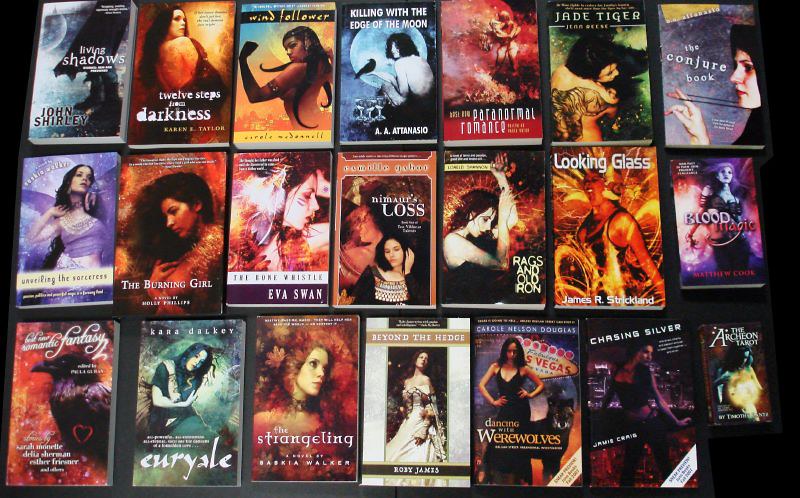The image displays an array of 21 fantasy and horror novels arranged in three rows on a black surface, with seven books in each row. The predominantly dark-themed covers feature gothic and emo aesthetics, showcasing primarily white women with black hair, along with occasional elements like birds and demonic figures. The books include titles such as "Living Shadows" by John Shirley, "12 Steps from Darkness," "Wing Follower," "Killing with the Edge of the Moon," "Paranormal Romance," "Jade Tiger," "The Conjure Book," "The Burning Girl," "The Lone Vestral," "Rags and Old Ron," "Looking Glass," "Blood Magic," "The Strangling," "Beyond the Hedge," "Dancing with Werewolves," and "Chasing Silver." The text on the covers is generally in white, complementing the dominant red hues and gothic imagery across the collection.